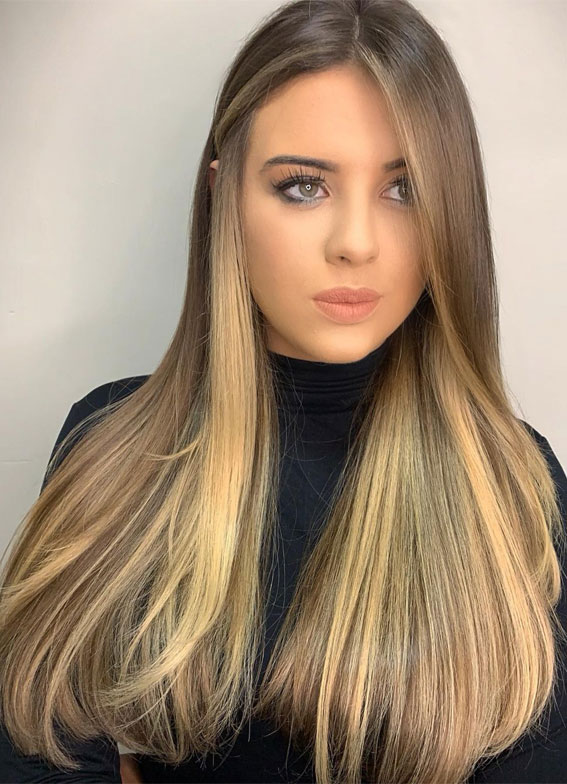In this detailed image, a young woman in her early to mid-twenties is shown facing the camera, possibly in a selfie or a photo taken by someone close to her. Her long, straight brown hair smoothly transitions into light blonde towards the ends, which drape over the front of her shoulders. Her face is accented with polished makeup, featuring dark, neatly groomed eyebrows, striking green eyes adorned with black and white eyeshadow, and heavy mascara that highlights her long lashes. She also has glossy pink lips, suggesting the use of lip gloss or lipstick. Dressed in a black turtleneck sweater with long sleeves, her overall appearance is that of someone who might be preparing to go out, giving off a vibe that is both poised and ready. Her expression is neutral, and although her gaze is directed slightly off to the side, there is an engaging quality in her look.